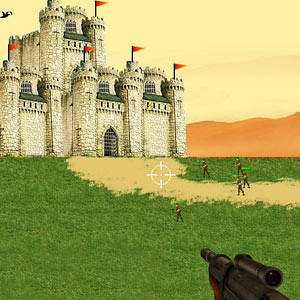This image, a piece of digital art from a video game, depicts a grand, medieval-style castle set against a pale yellow sky. The gray castle, adorned with darker gray rooftops, features several round turrets each topped with small, red, triangular pennant flags. There are five flags visible, all blowing to the right. The castle is positioned on a grassy hill, occupying the left two-thirds of the image's upper half. Visible along the horizon on the right side is an orange mountain range. 

Approaching the castle along a dirt path that leads to an arched doorway covered by a metal gate are five cartoon-like characters. These characters are walking through a lush green foreground. A sinister presence is hinted at by the sniper's rifle, visible in the lower right corner, pointed towards the castle’s entrance. The rifle is black with a red tip beneath the barrel, and it has a scope, suggesting the viewer's perspective within this first-person shooter game. White crosshairs hover over the tan pathway in front of the castle gate, further emphasizing the video game setting of the image.